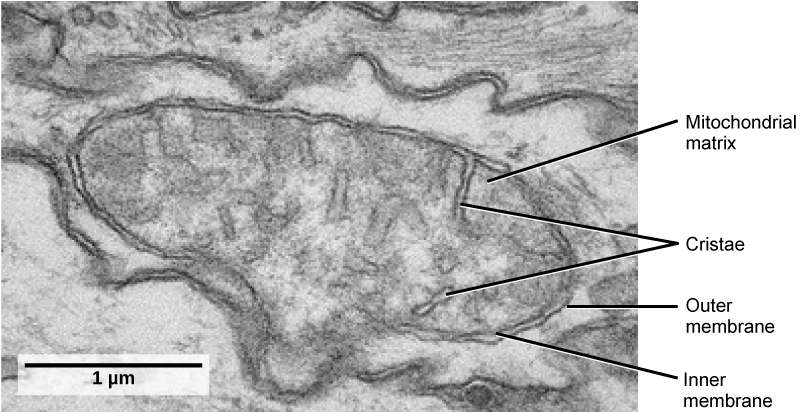This black-and-white image, appearing gray and blurry, seems to be a low-resolution, low-quality microscope image or possibly a pencil-drawn sketch displaying internal biological structures of a mitochondrion. Central to the image is an ovoid shape with various internal components labeled: the "Mitochondrial Matrix," spelled M-I-T-O-C-H-O-N-D-R-I-A-L, and "Cristae," spelled C-R-I-S-T-A-E, are identified with lines pointing to different parts within the ovoid. The outer edge is marked with labels indicating the "Outer Membrane" and "Inner Membrane." Below the image, on the bottom left corner, there is a black line with the text "1UM" written next to it, indicating a measurement reference.